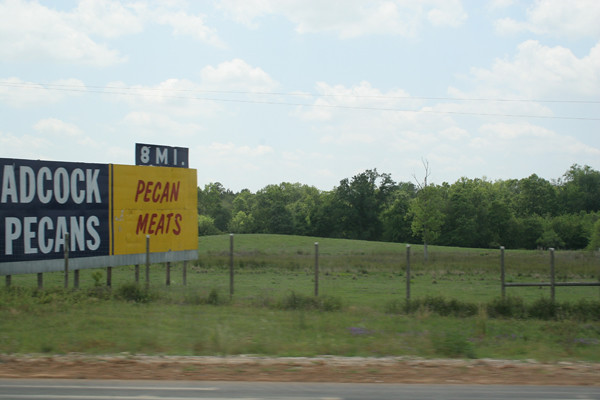In the photograph, a large billboard dominates a grassy field bordered by a fence. The fence's posts are clearly visible, leading the eye towards a lush expanse of green. Behind the fence, a second grassy field stretches out, gradually merging into a dense cluster of trees. Among these trees, one stands out starkly—its lifeless, leafless branches contrasting with the vibrant green foliage of its neighbors.

The sky above is a picturesque blue, dotted with numerous white clouds, adding to the serene rural atmosphere. The billboard, the focal point of the image, features two distinct sections. On the left-hand side, against a blue background, the text reads "Adcock Pecans" in bold white letters. The right-hand side of the billboard has a different design, with "Pecan Meats" written in red paint on a yellow background. Above this section, a smaller rectangular sign indicates "8 mi" (eight miles) in white lettering.

At the very edge of the photograph, a small segment of a road is partially visible, hinting at a path leading away from this idyllic scene.